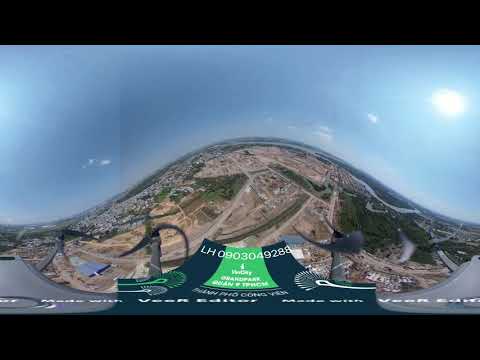This overhead image presents a detailed and intricate scene reminiscent of a video game screen, viewed from an airplane or drone. Central to the image is a prominent hill that rises from the ground, forming a natural focal point. This hill is surrounded by varied landscapes, including green patches of grass and brown areas, alongside clustered tiny buildings suggesting small cities at its base. To the left, the ground forms an upside-down triangle with more dense concentrations of buildings, possibly indicating a city. Adjacent to this triangular area is a vertical rectangular section of land. 

The upper portion of the image captures a blue sky, while the right side features something white, likely the sun. A distinctive element is the blue wing of the aircraft at the bottom center, bearing the white alphanumeric code "LH0903049288" and a green rectangle. The image is framed by a thick black border on both the top and bottom, enhancing the panoramic, bird’s eye perspective.